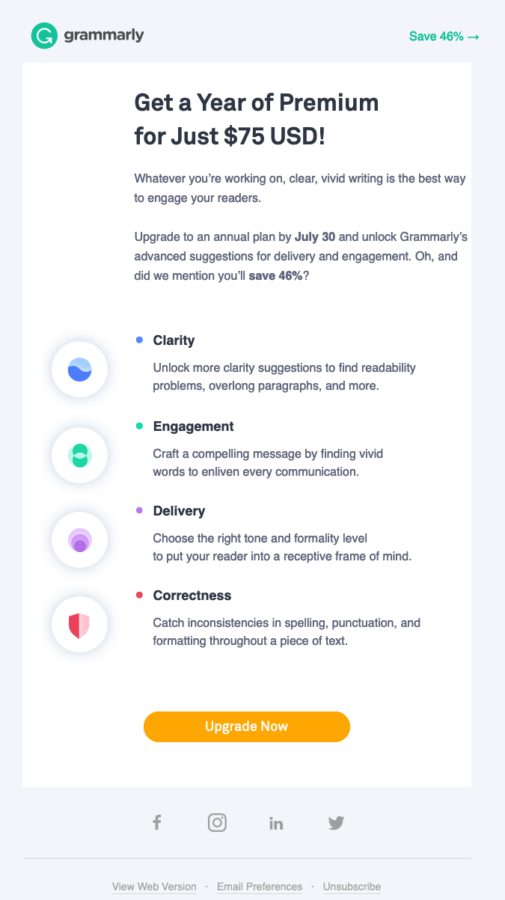The background of the image is light gray, with the central focus being a white rectangular section featuring various pieces of information. At the very top, there is the Grammarly logo, accompanied by a green circle containing a refresh button. Adjacent to this, there is a promotional offer highlighted with the text "Save 46%," followed by an arrow pointing to the right. This leads to the statement, "Get a year of Premium for just $75 USD!"

The message continues with a persuasive statement: "Whatever you're working on, clear, vivid writing is the best way to engage your readers. Upgrade to an annual plan by July 30," with the date emphasized in bold, "and unlock Grammarly's advanced suggestions for delivery and engagement." Additionally, the promotional offer is reinforced with the bolded question, "Oh, and did we mention, you'll save 46%?" 

Below this, four circles are sequentially labeled: "Clarity," "Engagement," "Delivery," and "Correctness," indicating the key areas Grammarly focuses on improving. At the bottom of the white rectangle, there is a yellow oval button with the text "Upgrade Now" in white. Finally, beneath this button are icons for Facebook, Snapchat, LinkedIn, and Twitter, suggesting the ability to share or connect via social media platforms.